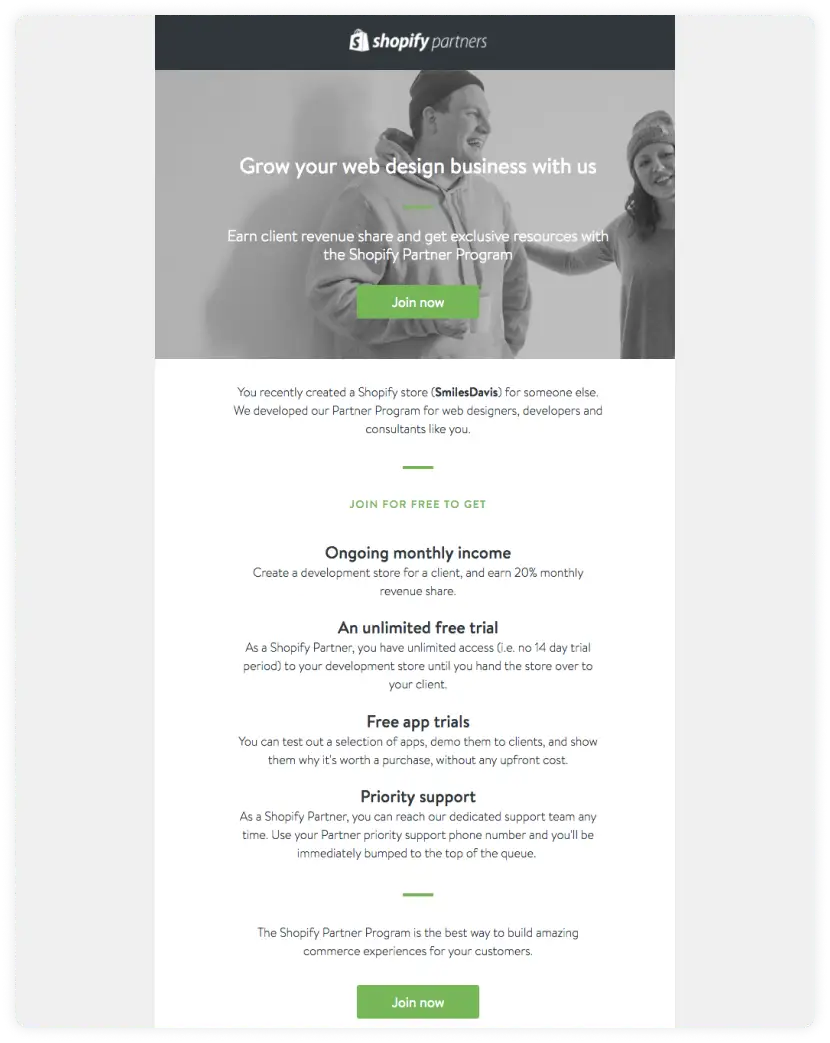The screenshot captures an informative advertisement for the Shopify Partner Program on a white background. It prominently displays a black box at the top, containing the text "Shopify Partners." Below, it reads, "Grow your web design business with us. Earn client revenue share and get exclusive resources with the Shopify Partner Program." A green "Join Now" button is clearly visible.

In the image, a man and woman stand side by side. The man is dressed in a hoodie and hat, while the woman, also wearing a hat, affectionately pats his arm. The scene suggests a moment of camaraderie and success. 

Another text snippet mentions, "Must be a winner," creating a positive connotation. It follows with, "You recently created a Shopify store. Smile, save us for someone else." The explanation continues: "We developed our Partner Program for web designers, developers, and consultants like you. Join for free to get ongoing monthly income. Create a development store for a client and earn a 20% monthly revenue share, with unlimited free trial."

The benefits of the Shopify Partner Program are then elaborated:

- **Unlimited Development Stores:** As a Shopify partner, you have unrestricted access to your development store until you transfer it to your client.

- **Free App Trials:** You can test and demo a selection of apps to clients without any upfront costs, showcasing their value.

- **Priority Support:** Gain access to a dedicated support team and a priority support phone number, ensuring you are bumped to the top of the queue for immediate assistance.

The caption reiterates that the Shopify Partner Program is the optimal way to build exemplary e-commerce experiences for your customers. The advertisement concludes with another green "Join Now" button, inviting viewers to take action.